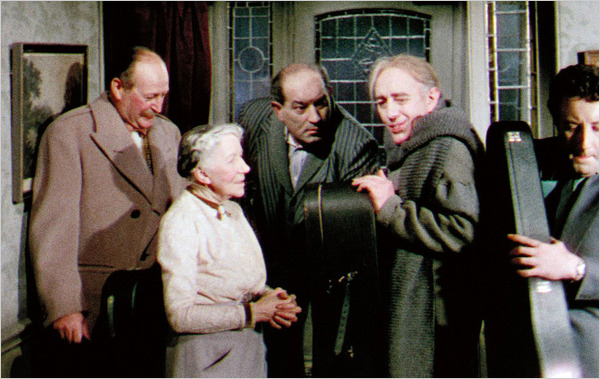This image, appearing to be a frame from an old movie or TV show set in the 1940s or 1950s, features a hazy, grainy aesthetic common to that era. The scene takes place in the entryway of an elegant house, showcasing an intricately designed glass door flanked by matching side panels and framed by heavy burgundy drapes. Five individuals are present in the frame. From left to right, there is a man in a brown wool jacket, looking downward, followed by an elderly woman with braided hair, dressed in a white dress, standing with her hands folded. Next to her is a man in a gray suit, slightly leaning forward. To his left, another man in a gray coat, smiling and holding a musical instrument case, and finally, a man on the far right, also looking down and holding a guitar case. The configuration and interaction suggest that they might be either arriving or departing, with the woman possibly welcoming or bidding them farewell. The background includes a wall with a partially visible painting, adding to the confined yet richly decorated setting.